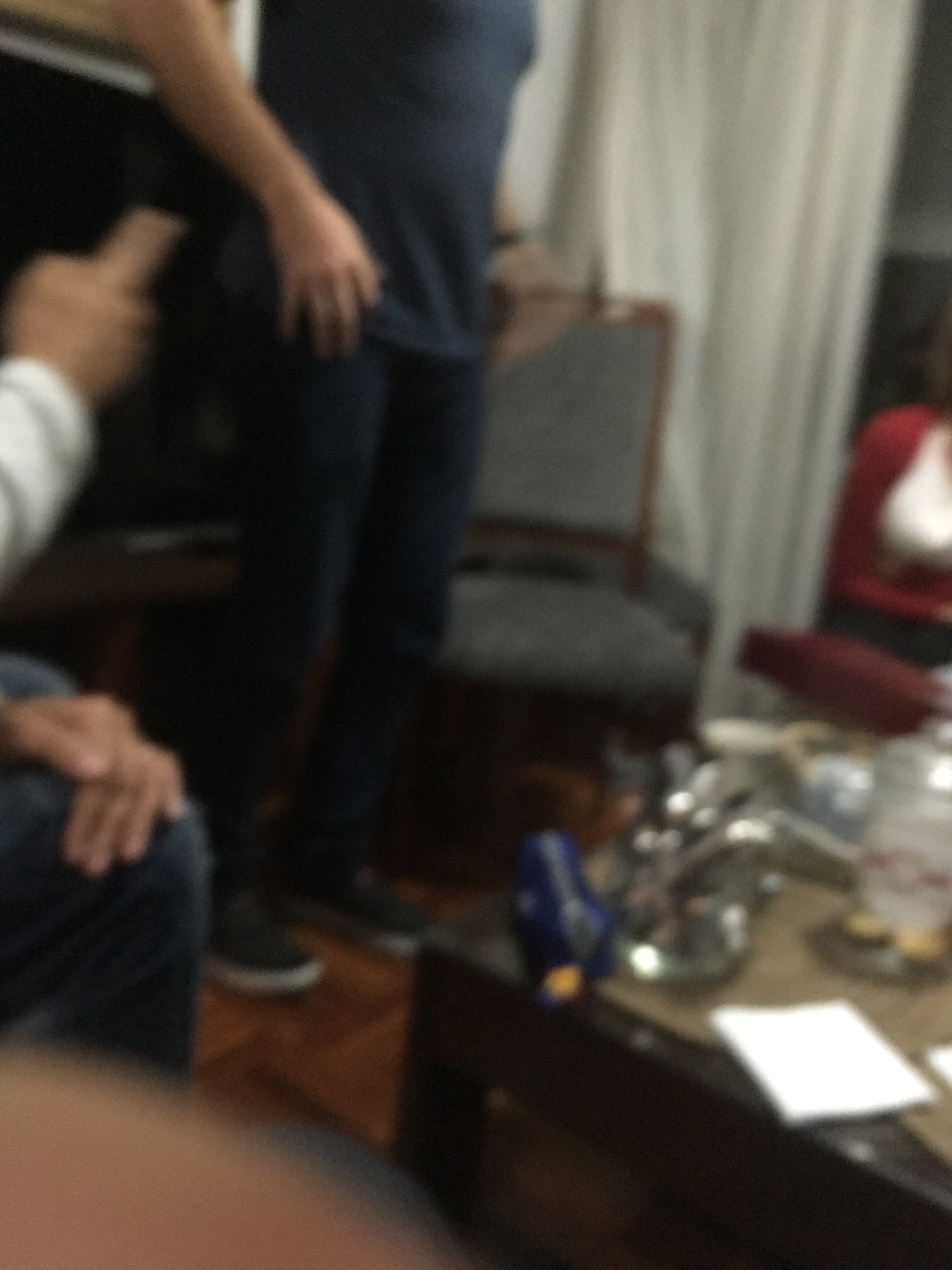In this blurry, portrait-oriented photograph, we see an intimate glimpse into someone's home. The image features two individuals, the focal points of the scene. The person standing on the right is dressed completely in blue, including blue shoes, blue pants, and a blue t-shirt. The photograph cuts off at about chest level for this person, obscuring their upper features.

To the right of the standing individual, another person is seated and partially captured. This person is observed with their left hand resting on their right knee, dressed in dark pants and a long-sleeved top, with only the sleeve on their right arm visible. The seated person appears to be shaking a finger at the standing individual, adding a dynamic and possibly conversational element to the scene.

The room itself has several key features: to the immediate left of the standing person is a chair, behind which a television is visible. Large white curtains frame the background, extending beyond the chair. In the foreground, a coffee table is cluttered with an assortment of items, hinting at the everyday life of the inhabitants. The overall atmosphere suggests a casual, lived-in space where a moment of interaction has been candidly captured.